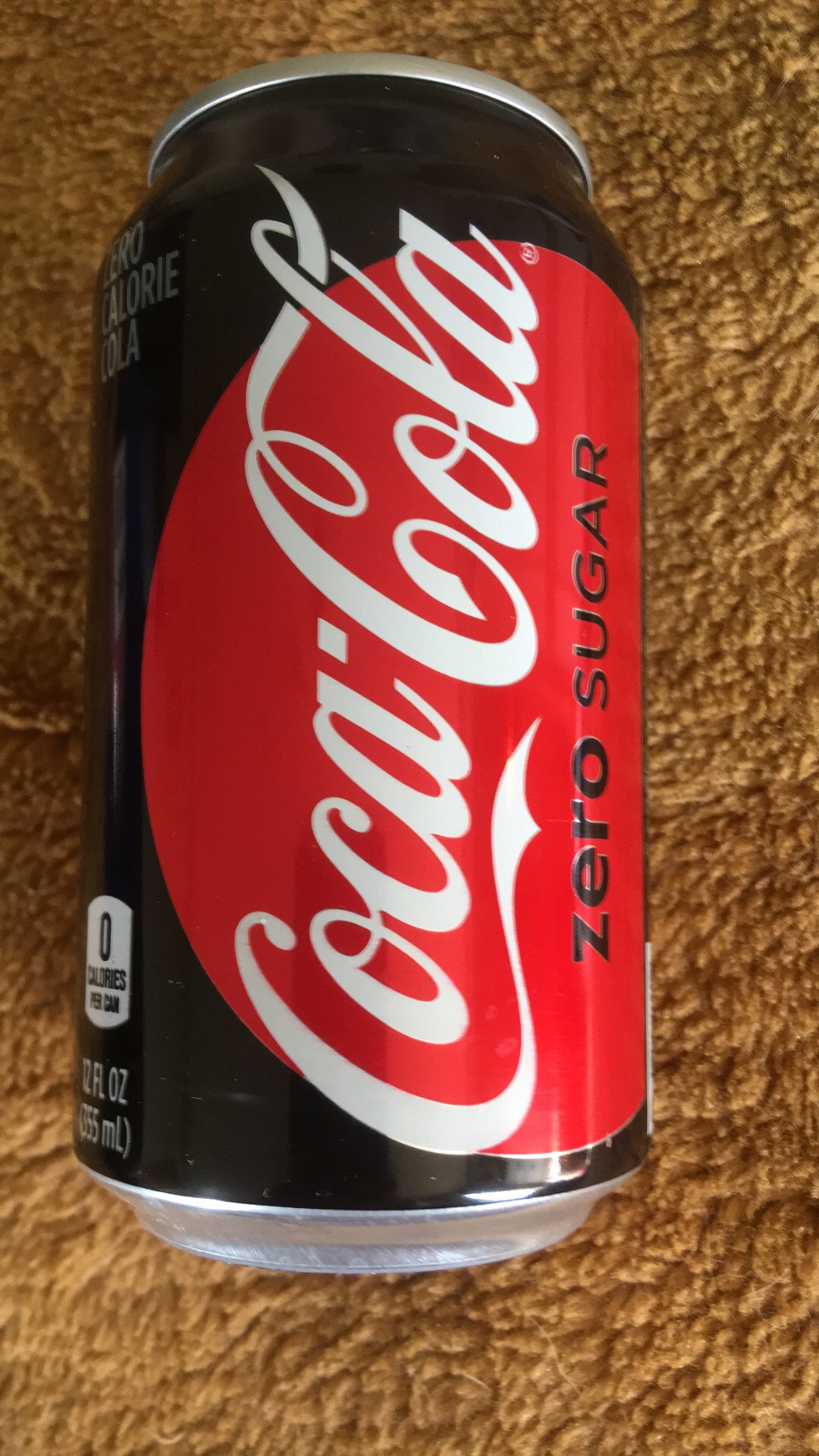The image is a close-up of a can of Coca-Cola Zero Sugar, lying on its side atop a soft, brown, low-pile carpet. The can prominently features the classic white Coca-Cola script running vertically over a large red circle, contrasted against the predominantly black design of the can. Notable text includes "Zero Sugar" and "Zero Calories per can" in black lettering underneath the Coca-Cola script. The can specifies its volume as 12 fluid ounces. The lighting from the right side of the image catches a slight reflection on the surface of the can, suggesting it is brand new.